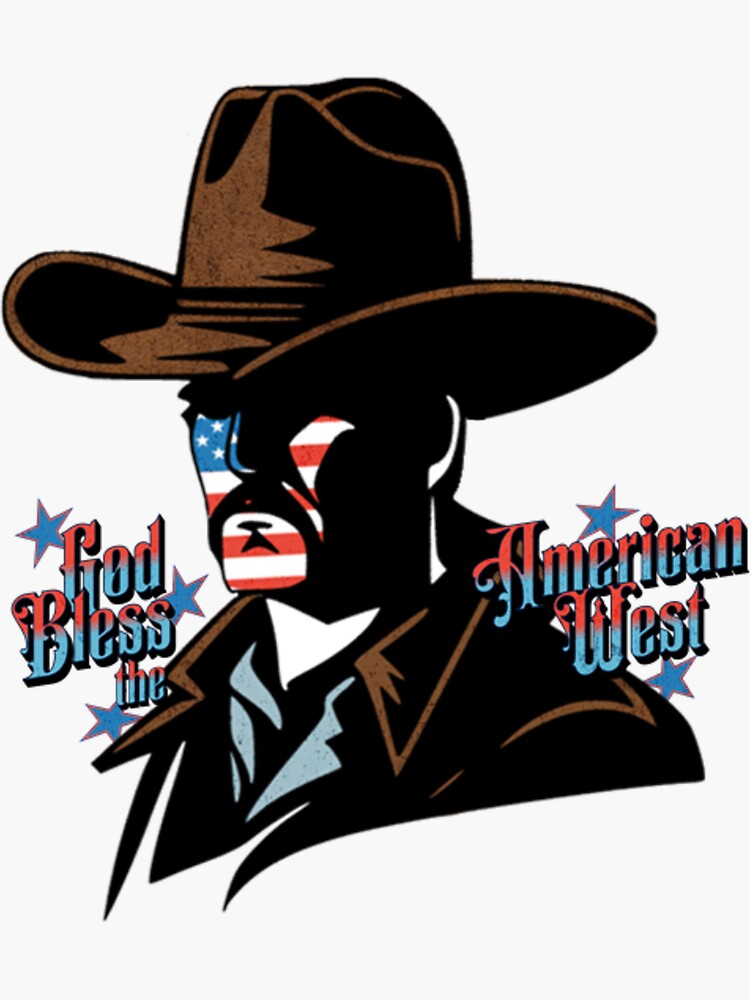This illustrated poster depicts a cowboy in a simple, stylized drawing, facing left at a 45-degree angle. He wears a wide-brimmed brown cowboy hat and a brown jacket with a visible collar. His face is covered in an American flag motif: the blue field with white stars occupies the area around his left eye, while red and white stripes extend across the right side of his face down to his chin. His eyes are not visible as his face is silhouetted in black, but the handlebar mustache is clearly depicted in black.

The poster features text on either side of the cowboy. On the left, it reads "God bless the," while on the right, it says "American West." The text has a gradient from red at the top to blue at the bottom, adorned with solid blue stars outlined in thin red. Specific stars appear as follows: one above the "E" in "American," one below the "S" in "West," one to the top left of the "G" in "God," one to the right of the last "S" in "Bless," and one below the "T" at the bottom. The background of the poster is white, which enhances the bold, patriotic colors in the illustration.